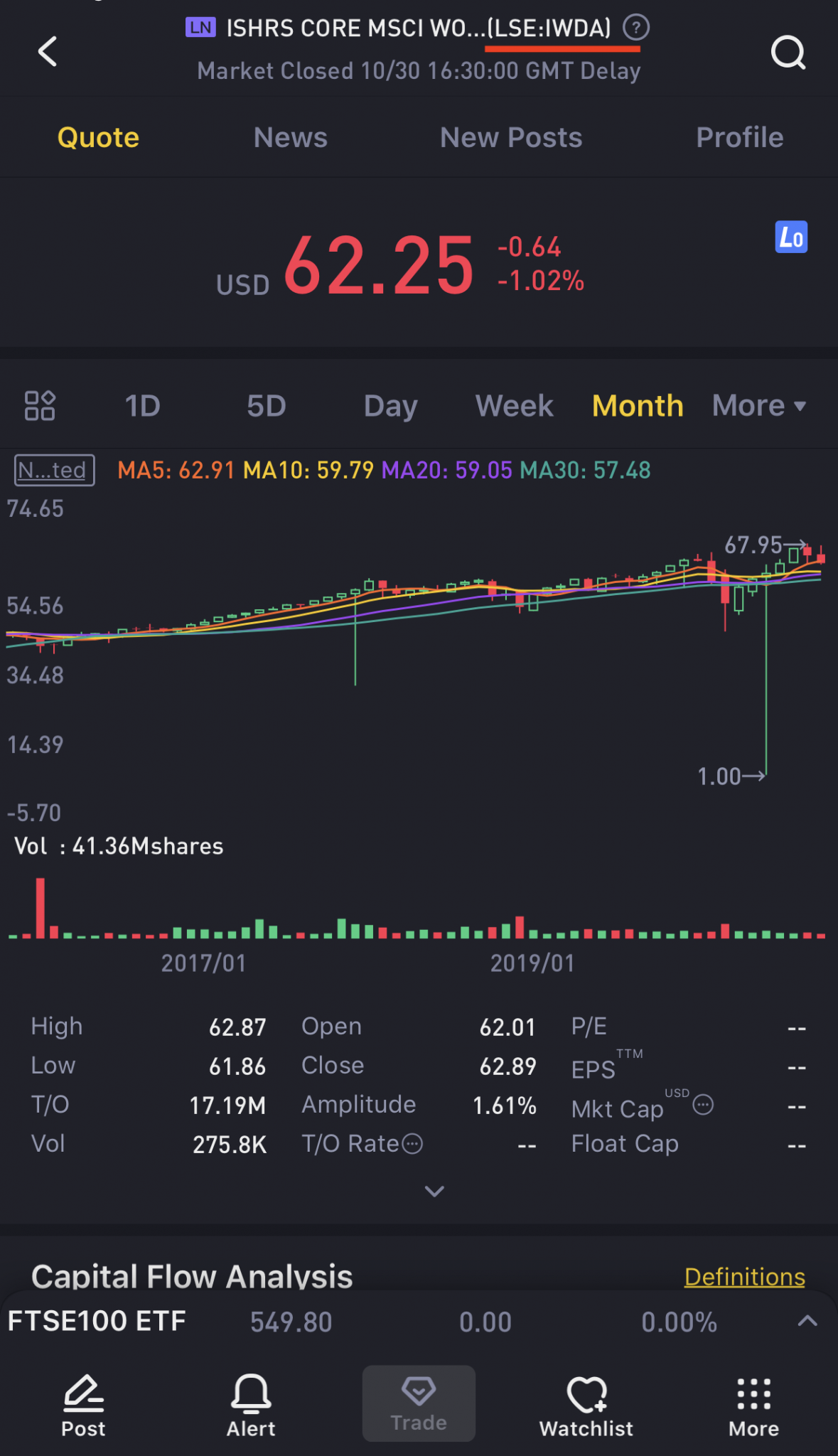This is a detailed screenshot of a stock quote page with a sleek, dark background. The screen features various elements in light gray, white, and other colors for clarity and emphasis. Dominating the center is a vibrant graph that illustrates the upward trend of the stock's price over time. 

At the top of the page, the header prominently reads "ISHRS CORE MSCI WO..." followed by market status text that notes: "Market closed 10:30, 16:30 GMT delay." Beneath this header is a navigation menu with options, including "Quote," "News," "New Posts," and "Profile."

In the middle right section of the screen, the stock price is prominently displayed in red at "USD 62.25," indicating that the price has decreased. Directly below this, the colorful chart showcases the stock's price movement over various periods, ranging from a single day to a month. 

Further down, another small bar graph in red and green provides additional insights. The dates of "January 2017" and "January 2019" along the x-axis help frame the long-term performance. The graph also includes markers for the stock's high and low prices during the selected time frame.

The layout and color scheme facilitate easy reading and quick comprehension for users monitoring the stock's performance.